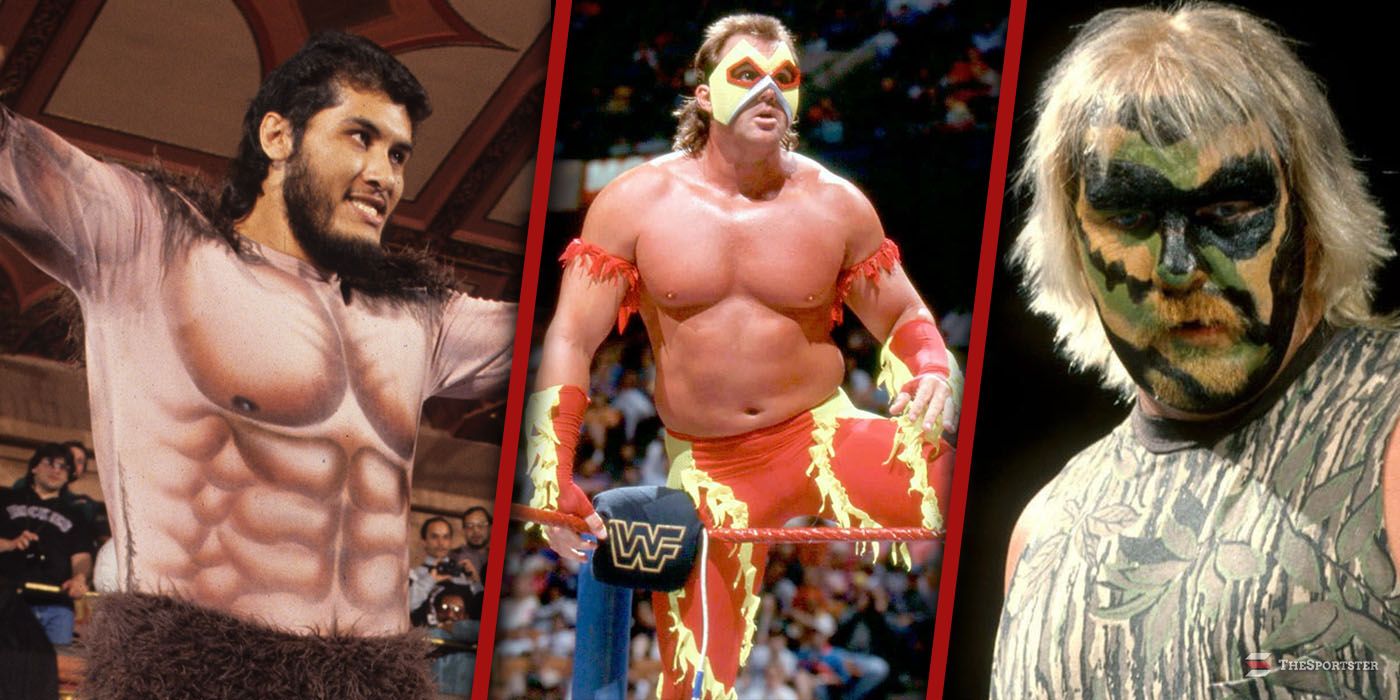This image features three distinct wrestlers from the 1990s, arranged side-by-side. The wrestler on the far left is sporting a fake abdominal shirt that displays a six-pack, paired with brown fuzzy pants. Positioned in the center, the second wrestler dons a striking outfit consisting of a yellow mask accented with an orange border around the eye area, along with red and yellow bands around his biceps, and matching flame-patterned gloves and tights. Completing the trio on the right is a wrestler clad in full camouflage gear, including a face painted in green, yellow, and black camo colors, alongside an army-style jacket. The vivid hues in this image range from tan, beige, and blonde to bright red, yellow, green, and black.